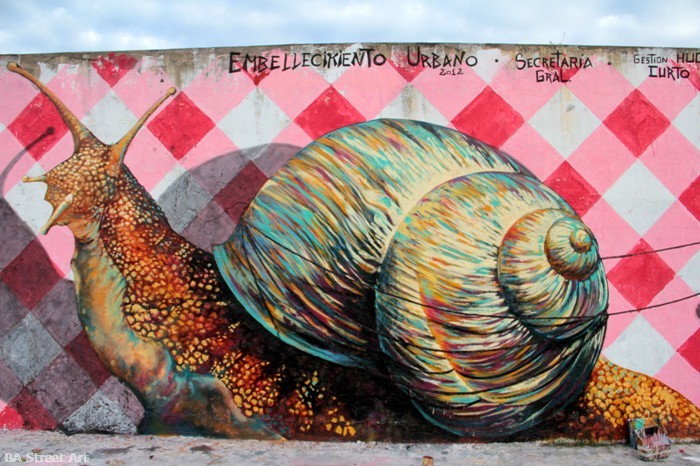This captivating mural, emblazoned on the side of a concrete wall, features a large, colorful snail. The snail stands out prominently against a vibrant backdrop of red, white, and pink checkered patterns, reminiscent of a tablecloth. The intricate details of the snail’s enormous shell, which swirls with a spectrum of colors including purples, yellows, blues, and greens, are beautifully rendered, showcasing its curves and lines with meticulous precision. The snail itself, painted in shades of brown with two antennae, is facing to the left. Above the striking imagery, Spanish text reads, "M. Bellicanto Urbana 2012 Secretarial Graalgestion Heliocurto." Below, at the base of the mural, art supplies or possibly litter can be seen scattered on the pavement. Bright and imaginative, this artwork breathes life into the concrete, inviting observers to marvel at its detailed and colorful depiction.